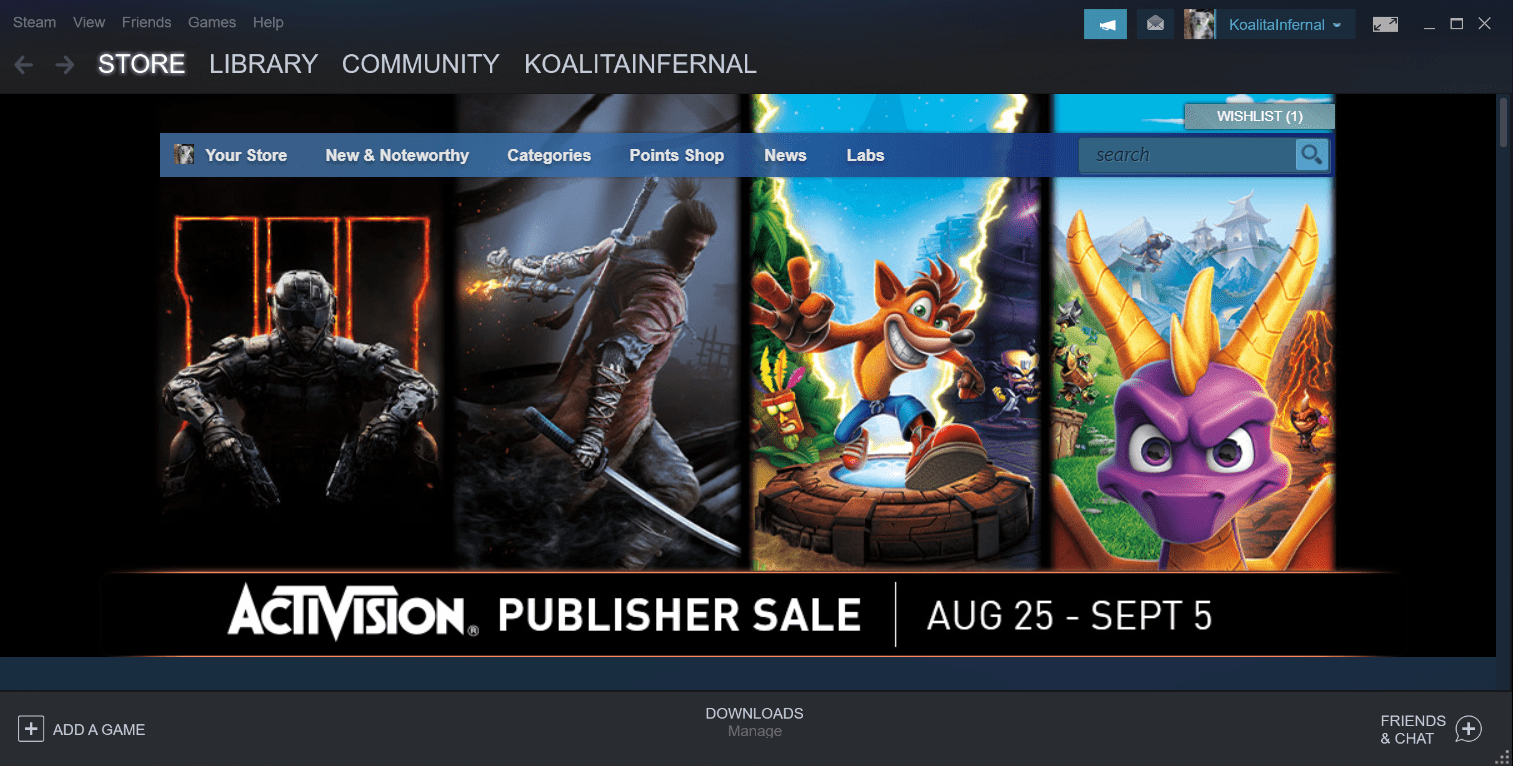The image displays the Steam Store website interface, featuring a predominantly black background with dark gray borders on the top and bottom. 

Starting from the top left, the Steam logo is situated in lighter gray, followed by menu options: View, Friends, Games, and Help. On the top right, there's a blue button with a left-facing arrow icon, adjacent to a mail icon. Next to the mail icon, there's a small profile picture of a koala, indicating the user's profile named "Koala Rain Mail" in blue, accompanied by a gray down-facing arrow. Further to the right, there is a gray button with dark gray diagonal arrows, and at the far right are the Minimize, Maximize, and X buttons.

Below this top section, on the left, there are left-facing and right-facing arrow buttons in light gray. To the right of these arrows, the word “Store” appears highlighted in white, while the subsequent options—Library, Community, and K-O-A-L-I-T-A-I-N for F-E-R-N-A-L—are in light gray.

Directly beneath this navigation bar, there is a row of thumbnail images: starting from the left, a Halo military officer, followed by an anime character holding a sword, then a fox jumping over a well, and finally, a purple-headed dragon on the rightmost position.